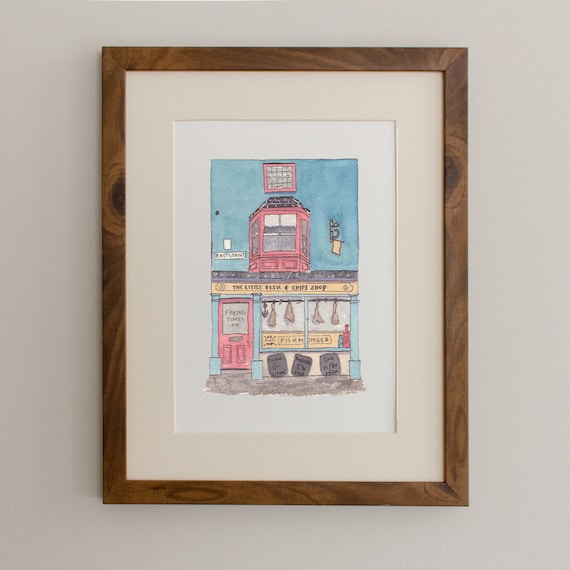In this detailed artist's colored pencil drawing, framed in medium-toned wood with visible knots, hangs on a gray wall. The wooden frame holds a layered matting; an outer off-white mat and an inner white mat framing the artwork. The picture depicts the front of a whimsical and brightly colored butcher shop. The butcher shop features a prominent blue exterior with a slanted tiled roof, a pink bay window, and a red door. The shop's windows showcase various meats hanging, and the glass pane of the door bears the etched words "Frying Times." A yellow banner underneath reads "The Eerie Fish and Chip Shop." The scene is further detailed with three barrels outside the windows, possibly serving as seats or signs to advertise meats inside the shop. Topping the building is a striking red structure resembling a crow's nest, giving the impression of a lighthouse, adding a unique charm to the folk or naive art style of the illustration.